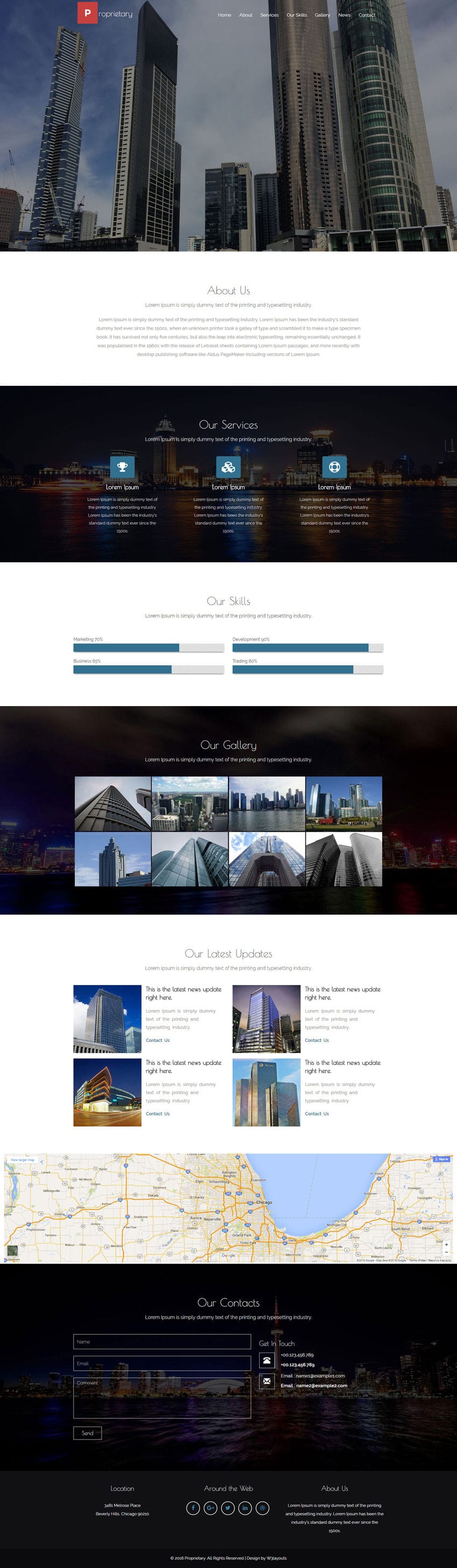This image depicts a composite screenshot of a website, displaying each webpage in a continuous vertical sequence. At the top, the website showcases a banner extending from left to right, featuring a white menu bar and a photograph capturing an upward view of buildings. Beneath the banner, the "About Us" section follows, presented on a plain white background. Next in line is the "Our Services" section, succeeded by "Our Skills" and, subsequently, the "Gallery" section. The layout allows one to visually browse through the entire website by scrolling down, offering a comprehensive view without the need to click on individual links.